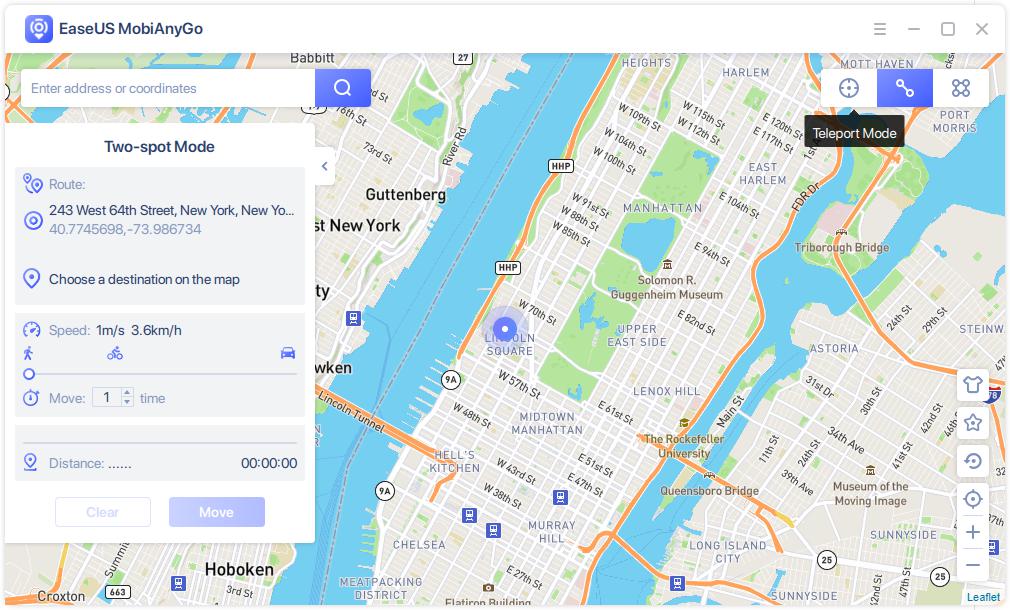The image portrays a detailed map interface, seemingly centered on a section of New York City. In the upper left corner, there is a user-friendly search bar labeled "Enter an address or coordinates," allowing users to input specific locations seamlessly. The map indicates a search or a route leading to 243 West 64th Street, New York, NY. Displayed coordinates are 40.7746698, -73.986734, and users can choose destinations on the map, with movement speeds shown in different units (1 mile/s and 33.6 km/h). Additionally, the interface features a button with a black information bubble labeled "Teleport Mode." The map itself utilizes a color palette primarily consisting of blue, brown, green, black, and gray, though no specific landmarks are identified in the immediate view.